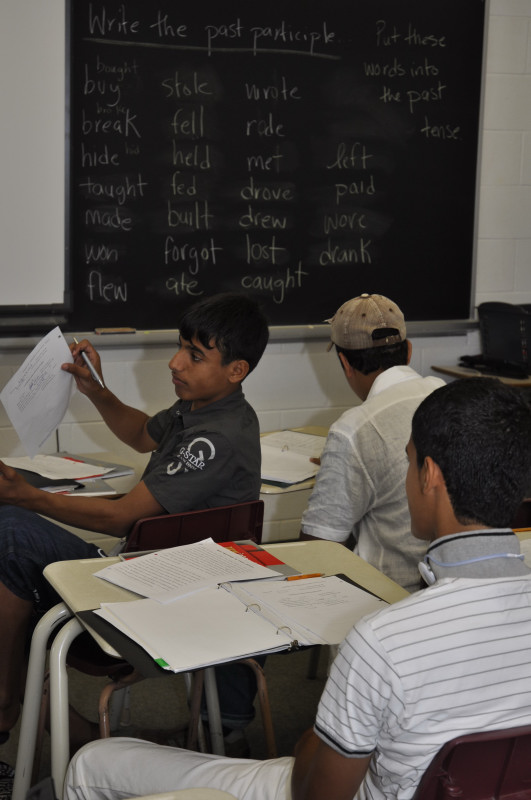The image depicts an indoor classroom setting with a carpeted floor and several desks arranged at the bottom. At the center of the image, three students sit facing away from the camera, suggesting their attention is directed towards a teacher out of the frame. The student closest to the camera wears a gray short-sleeved shirt, blue jeans, and is holding a pen and papers while looking to his left, possibly interacting with someone. Behind him, another student in a white top with a brown hat is looking down at his notes, while the third student, also in a white shirt, is focused on writing in his open notebook. The chalkboard at the top of the image features instructions written in chalk, prompting students to "write the past participle" and "put these words in the past tense," listing words such as buy, break, hide, taught, stole, fell, held, built, rode, ride, paid, wore, drunk, drank, write, met, left, fed, drove, mace, drew, forgot, lost, and caught. The colors throughout the image include various shades of off-white, white, black, gray, brown, tan, red, orange, and yellow, reinforcing the typical academic ambiance.